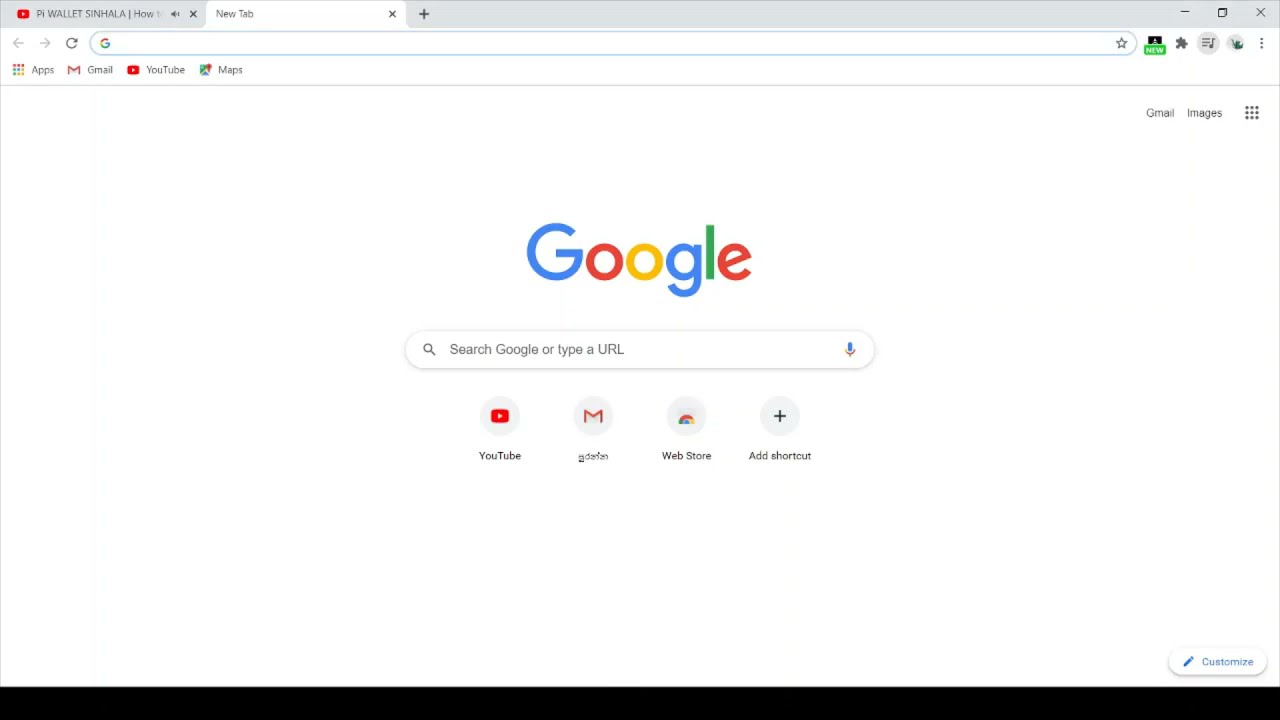The image depicts a computer screen displaying a web browser window open to the classic Google homepage. The Google logo, presented in its distinctive multicolored letters—blue "G," red "o," yellow "o," blue "g," green "l," and red "e"—is prominently centered. Below the logo, the search bar reads, "Search Google or type a URL." Underneath the search bar, there are four shortcut icons: YouTube, Gmail, the Web Store, and an option to add a shortcut.

At the very top, the browser shows two tabs: the active tab, labeled "New Tab," and an adjacent tab with the YouTube logo, which is not open and contains a title too small to decipher. Notable browser interface elements include the address bar, various control icons for extensions, and typical Chrome features. In the upper right corner, icons for Gmail, Google Images, and the app selection grid are visible. Additionally, the bottom of the screen features a black bar with a “Customize” button located at the bottom right corner.